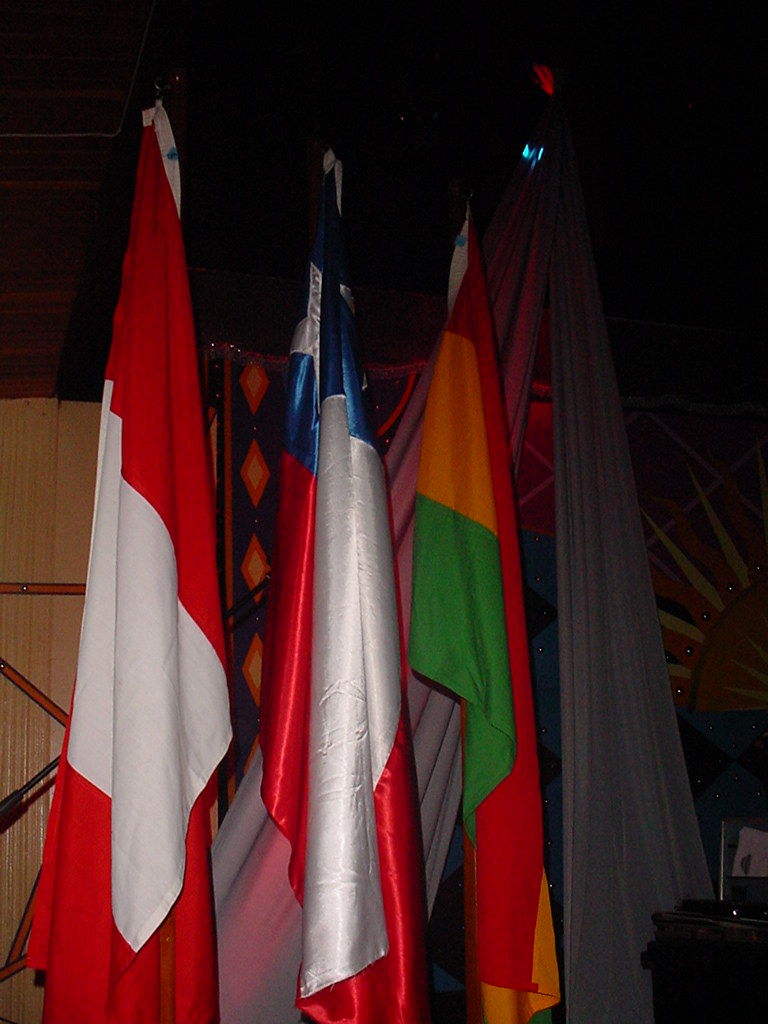This photograph captures a row of flags on flagpoles set in an indoor environment, all drooping without the aid of wind. The most leftward flag is divided equally into three vertical sections of red, white, and red. Adjacent to it is another flag with horizontal bands of white, red, and blue, featuring a prominent white star in the blue section. The third flag displays a vertical tricolor of green, orange, and red. The background is dominated by a gray curtain hanging from the ceiling in a triangular layout, with an overhead light casting illumination onto the flags below. Although the flags are not easily identifiable due to their folded state, this detailed scene suggests an organized display possibly representing different entities or nations.